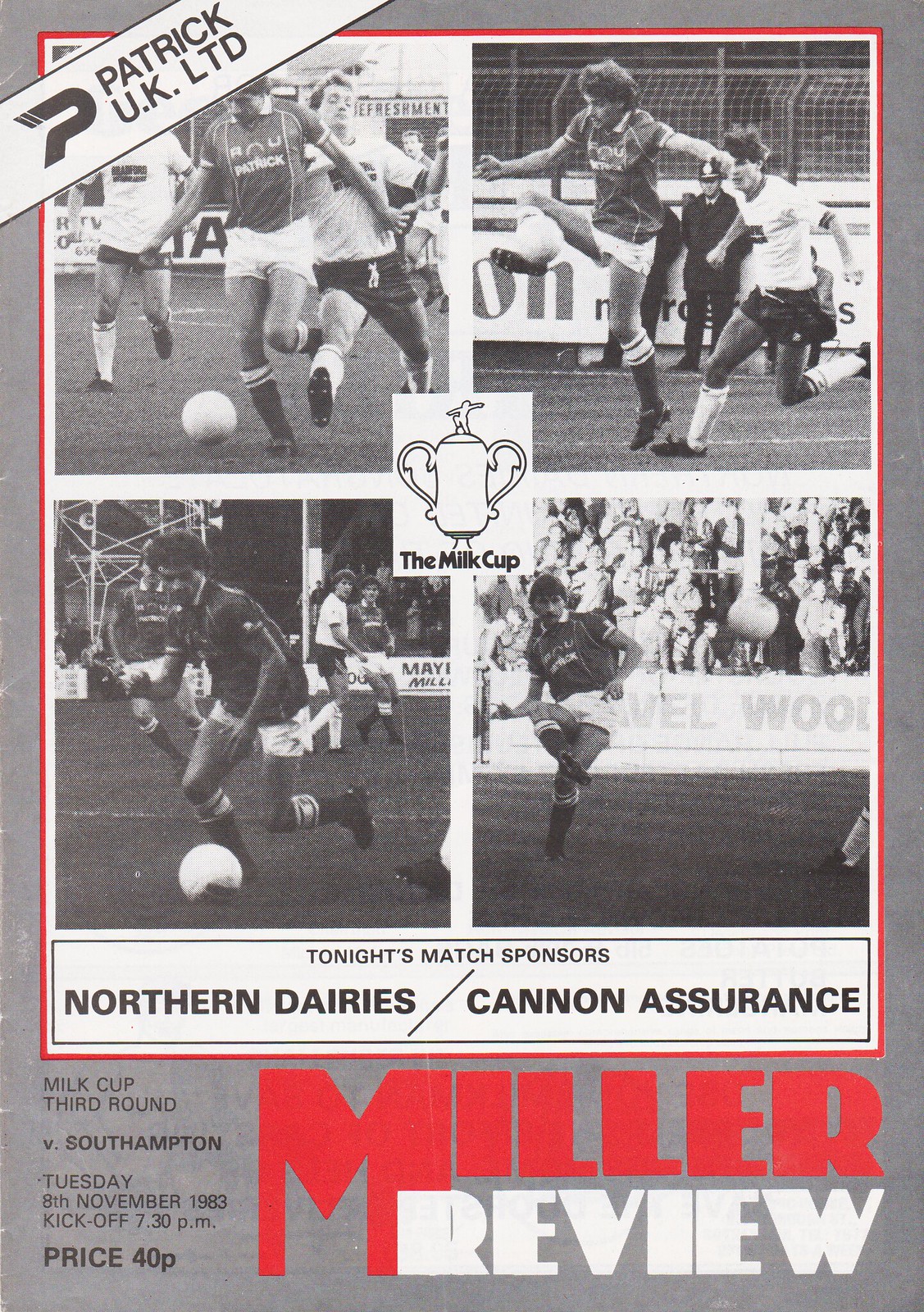This black and white image, framed by a thin red border, serves as the front cover of the Miller Review program for the Milk Cup. Dominating the design is a central collage consisting of four black and white photographs, each depicting men playing soccer. Nestled in the middle of this collage is an illustrated outline of a trophy, labeled "The Milk Cup." Above these images, in a white banner with a gray border, the text "Patrick UK LTD" is prominently displayed. 

Directly beneath the photographic collage, the caption reads "Tonight's match sponsors," flanked by "Northern Dairies" and "Cannon Assurance." Further down on the left, the details of the match are provided: "Milk Cup 3rd Round V Southampton, Tuesday 8th November 1983, kickoff 7.30pm, price 40p." On the bottom right, in striking letters, the title "Miller Review" is presented, with "Miller" in red and "Review" in white. The lower right corner is visually anchored by this same red lettering.

The contrasting uniforms of the soccer players in the photos—some in darker jerseys with white shorts and others in lighter jerseys with dark shorts—add dynamic visual interest, despite the monochromatic scheme.